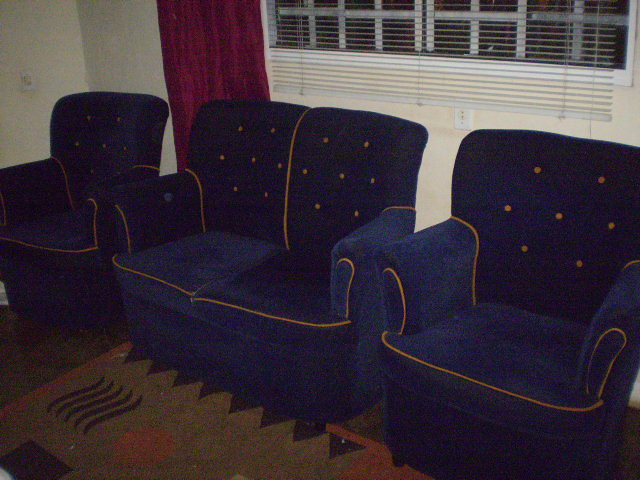This is a color photograph taken indoors, showcasing a group of two plush chairs and a matching loveseat arranged beneath a window. The furniture is upholstered in dark navy blue velvet with distinctive orange or gold piping along the edges and orange or gold buttons embellishing the backs of the seats, arranged with two at the top, three in the middle, and two at the bottom. The walls are cream-colored and feature a large window with white pull-up blinds that divide the view into rectangular panes. On the right side of the window, a rich burgundy curtain, drawn back, adds a touch of elegance to the scene. Underneath the furniture lies a brown, tan, and orange area rug with a geometric pattern, characterized by a zigzag outer border in black and some black wave designs along one edge, suggesting it could be made of wool. The overall setting exudes a cozy and sophisticated ambiance.